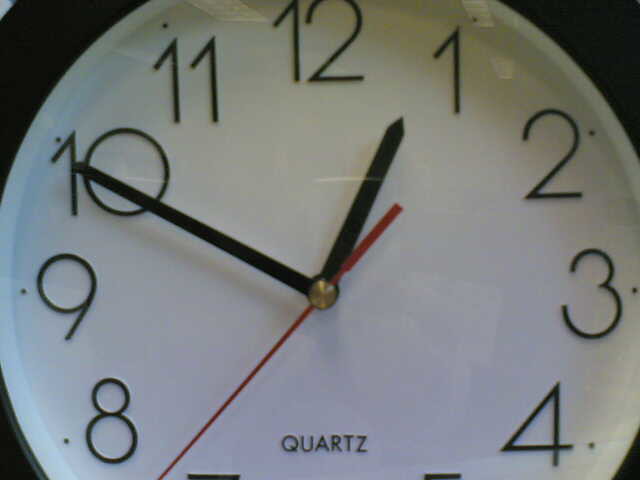This photograph captures an analog clock, though it appears slightly out of focus due to significant zoom. The white clock face, adorned with black numerals, dominates the image, with portions extending beyond the frame's edges, suggesting a very close-up shot. The clock features a black hour hand and a black minute hand, contrasted by a slender red second hand, all anchored centrally by a small, brass or golden-colored hub. At the bottom of the clock face, the word "quartz" is inscribed in black letters. The dark border of the clock is faintly visible in the corners of the photograph, with no other details discernible in the background.